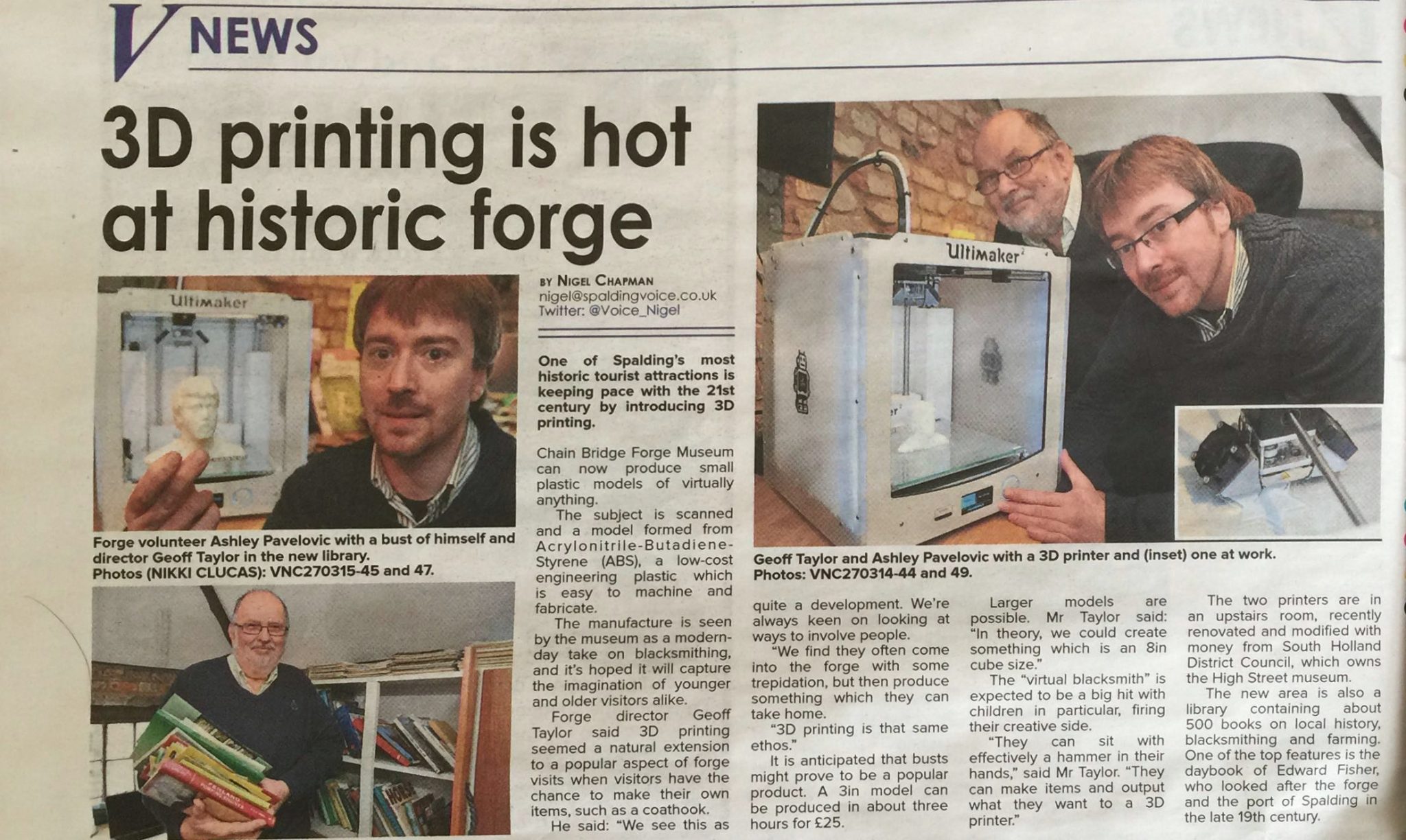An online newspaper page, shaded in gray tones, prominently features "V News" in bold black text at the top left corner, underlined by a horizontal divider. Below, a striking headline in large black letters reads, "3D Printing is Hot at Historic Forge." The article is authored by Nigel Chapman, whose contact information includes both his email (ending in .co.uk) and his Twitter handle. 

Accompanying the article, an image depicts Forge volunteer Ashley Pavlovich holding a white bust, identified as a sculpture of himself, alongside director Jeff Taylor in the new library. The photograph credits go to Nicky Klukas, labeled with reference numbers VNC 270315-45 and 47.

Further down, another image features a middle-aged bald man with glasses and a slight beard, dressed in a black long-sleeve sweater. He is holding a stack of folders and books, set against a background filled with more books, suggesting a library or academic environment.

In the top right corner, a photograph showcases Jeff Taylor and Ashley Pavlovich standing beside a white mechanical apparatus with a glass front, clearly showing the white busts being produced within. The caption identifies the men and describes the device as a 3D printer, mentioning additional photo reference numbers VNC 270315-44 and 49, indicating one image shows the printer in action.

The comprehensive article spans the length of the page, detailing the ongoing advancements and applications of 3D printing technology at Historic Forge.